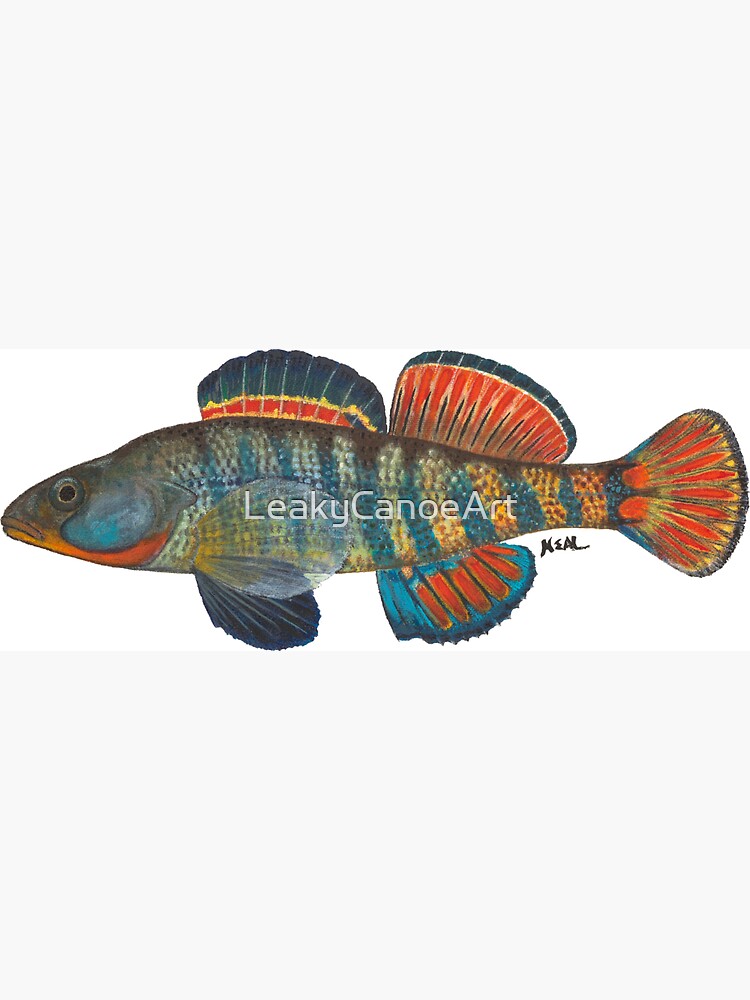The image features an artistic depiction of a rainbow darter fish against a white background. The fish is horizontally oriented with a predominantly green body that transitions into yellow stripes near the tail. The tail fin showcases vibrant red coloring with hints of blue and yellow, while the top fins are notably large and fan-like, composed of greens, bright reds, blues, and yellow streaks. The bottom fins start green and become transparent. Notably, one of the top fins is predominantly green with a red stripe bordered by yellow, and the other upper fin is blue and red, creating a striking visual contrast.

The fish’s body displays an intricate pattern with streaks of dark blue, light blue, and interspersed yellow. Its head, facing left, features blue shading with a red underside and black eyes. The tail presents a flame-like appearance with layers of reddish-orange, yellow, and hints of blue.

The painting, likely rendered in acrylic, sits on a vertically aligned rectangular background. There is a signature reading "Keel" or "Keir" near the fish’s tail in black lettering, and a watermark across the fish that reads "Leaky Canoe Art" in white lettering, providing an additional layer of authenticity and artist attribution.